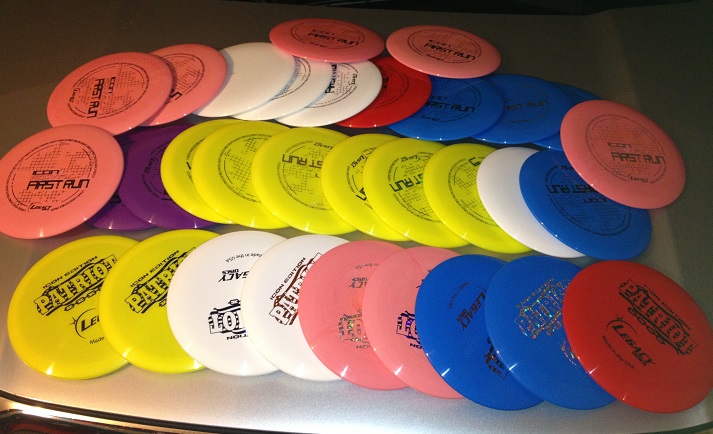The photograph, likely taken indoors with a flash and possibly on an iPhone given its slight overexposure and lack of sharp focus, depicts a collection of frisbees spread across a white surface. The background, especially in the top left and top right corners, is poorly lit, causing the edges of the white surface to fade into darkness. The frisbees are haphazardly arranged, stacked and partially overlapping each other. 

There appear to be around 25 frisbees, organized in three loose rows. The frisbees come in various colors: several are yellow, white, salmon (or pink), two are deep purple, two bright red, and six vibrant blue. Many of the frisbees are adorned with writings and logos, with recurring words such as "Patriot," "Legacy," and "First Run." Specific details are visible on some, for instance, a red frisbee features the word "Patriot" with a chain link under it and the word "Legacy" beneath. Despite the scattered arrangement, these discs seem ready for use or to be picked up by someone.